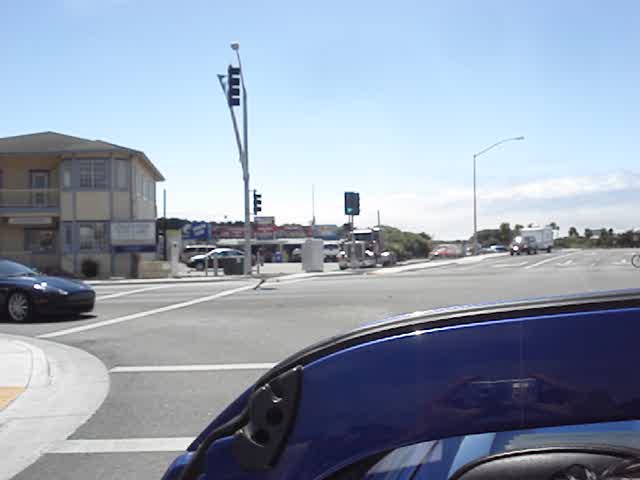A vibrant and detailed photograph captures a busy intersection drenched in bright, clear sunlight. The sky above is a vivid blue, adorned with white clouds. From the perspective of the image, it appears to be taken from a motorcycle due to the visible black and deep blue visor in the shot. However, it could also be from a convertible, wherein the driver's reflection is visible in the visor.

In the middle of the intersection, traffic lights direct the flow of numerous vehicles. To the left of the image, a black car is entering from an adjacent street, while an SUV can be seen pulling a trailer across the way. On the right side of the image, a large semi-truck is parked. 

The road is wide, featuring multiple lanes, including two lanes for straight travel and one for a right turn. Arrows on the pavement guide the vehicles. A yellow, two-story wooden building with a beige sign (unreadable from this distance) is situated to the back-left, suggesting a commercial area. Surrounding the buildings are a few trees, adding a touch of green to the urban scene, and numerous smaller signs, perhaps indicating a nearby parking lot.